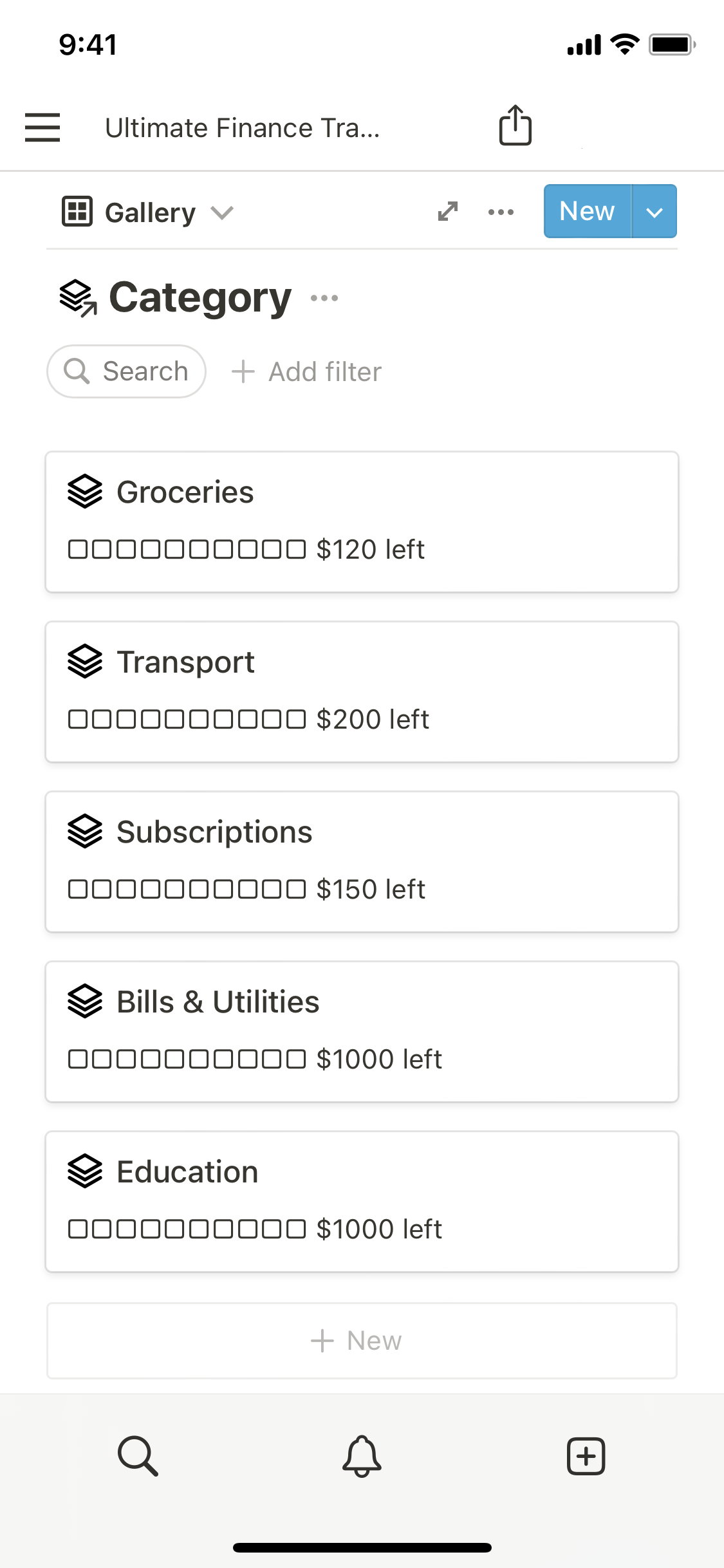This screenshot captures the interface of "The Ultimate Finance Track," a mobile app dedicated to finance tracking and management. The time displayed is 9:41. At the top of the screen, there is a menu icon on the left and a share icon on the right. 

The primary section showcases a title labeled "Category," with a search bar below it and an option to add filters, enhancing the user experience by allowing easy navigation and customization. A prominent "New" button is visible for users to add new financial entries seamlessly.

Various categories are displayed, each with its respective budgets and remaining amounts: 
- Groceries: $120 left
- Transport: $200 left
- Subscriptions: $150 left
- Bills and Utilities: $1,000 left
- Education: $1,000 left

Each category features a progress indicator illustrating the spending relative to the allocated budget, helping users quickly assess their financial status in different areas.

In the footer section, there are icons for search, notifications, and adding new entries, facilitating rapid access to essential functions. The interface is designed to be clean and organized, making it user-friendly for tracking spending across multiple categories efficiently.